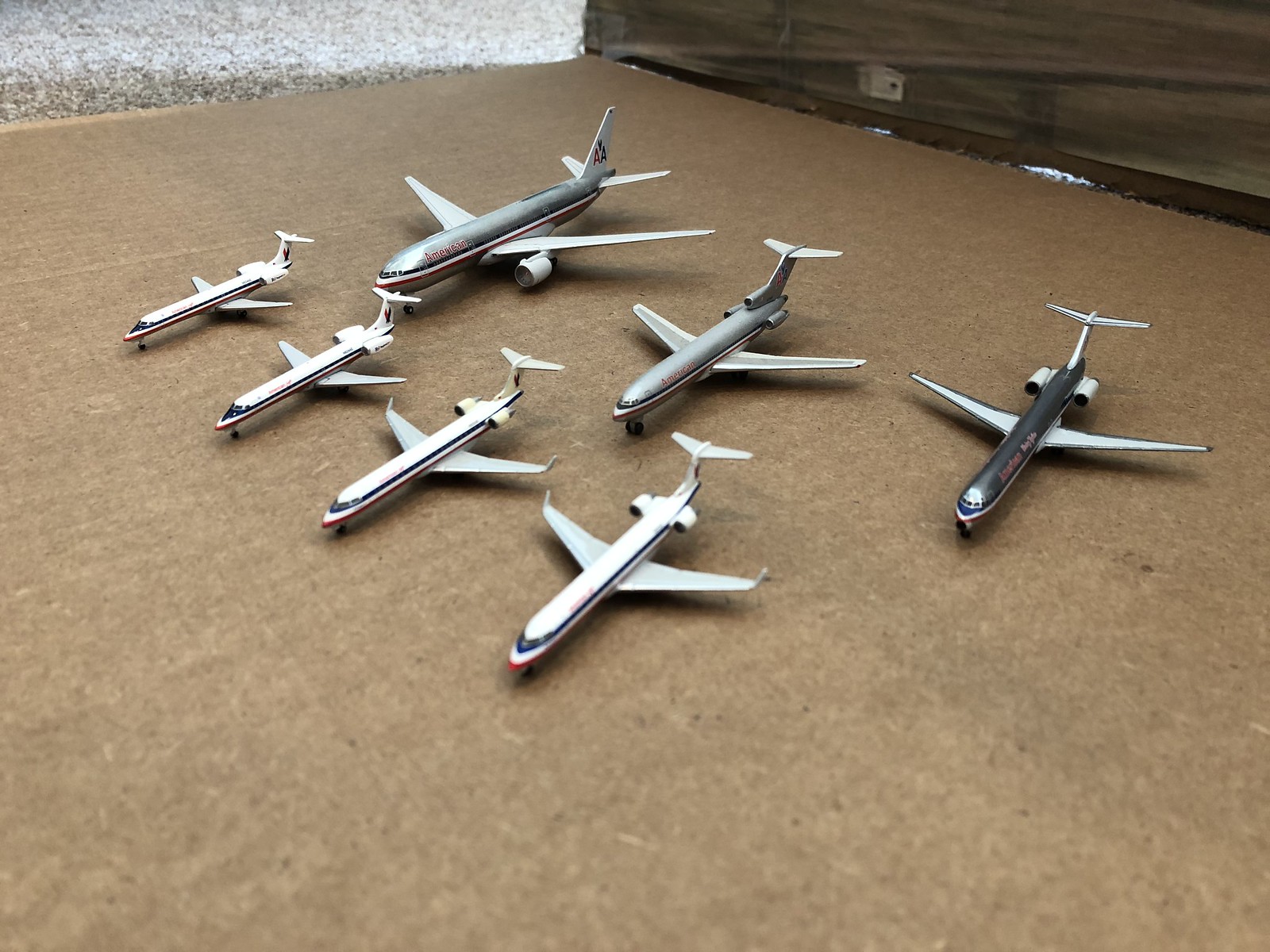The image showcases seven scale model airplanes meticulously arranged on a piece of cardboard, set against a background featuring fuzzy gray carpet in the top left corner and a wooden object to the top right. The models are lined up in two aligned rows, with four smaller planes in front and three larger ones in the back. 

The front row consists of four identical, white-bodied planes, each adorned with dark blue, white, and red stripes. These planes are uniform in design, featuring twin rear-mounted engines and large wings with upturned tips. Their noses are aligned diagonally towards the lower left corner of the photo.

In the back row, the planes vary in size and design, all primarily silver with accents of blue, white, and red. The plane furthest to the left is the largest, resembling a commercial jet with two large engines suspended from the inner portion of its wings. The middle plane, slightly smaller, has twin engines plus an additional engine mounted at the top of the tail fin. The rightmost plane is a slender model with a darker gray body and twin engines mounted on the rear. These details suggest the planes might represent different aircraft from the American Airlines fleet, hinted by the noted red, white, and blue color scheme and potential "AA" markings observed on one of the tails.